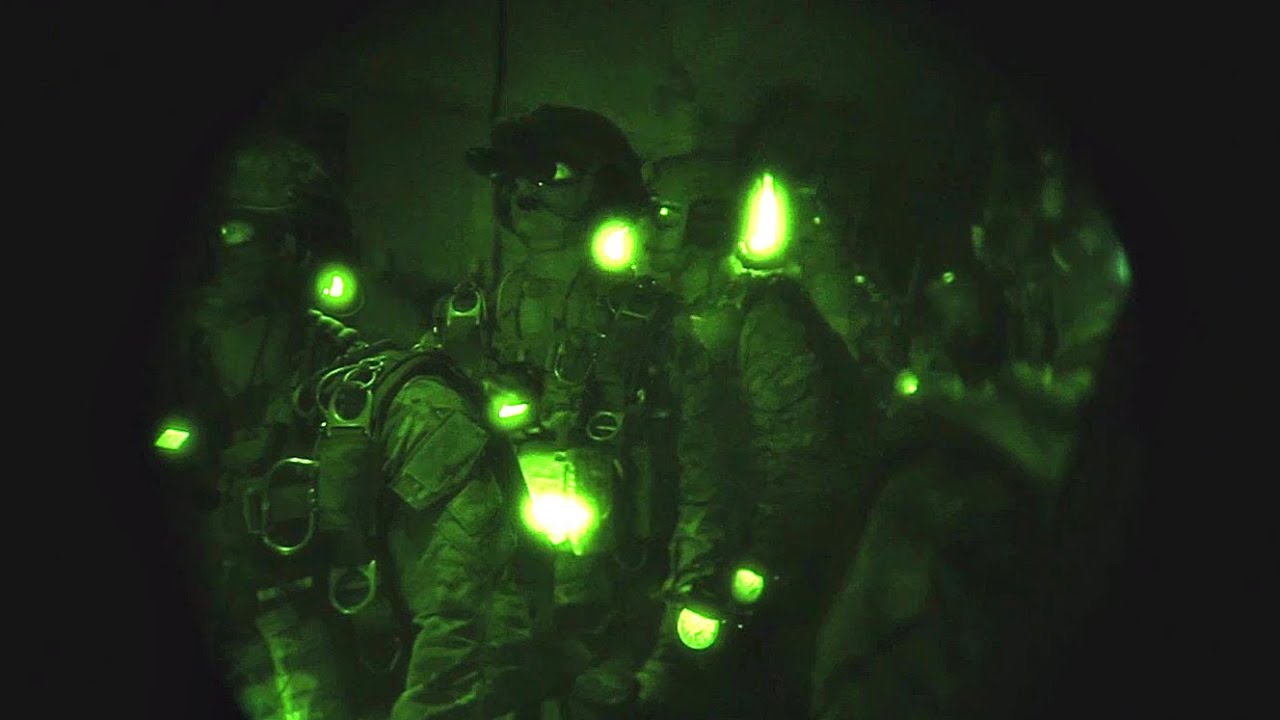This image depicts a group of individuals in a dimly lit environment, likely captured through night vision, with a greenish-yellow tint dominating the scene. It features four people, dressed in dark greenish-gray military or tactical uniforms, complete with helmets, night vision goggles, and harnesses. There are several bright areas in the image, particularly white with a green outline, which appear as reflections from their equipment, possibly flashlights mounted on their wrists or shoulders designed to be visible only through night vision. The setting seems to be a dark, enclosed space, such as a building or cavern. Notably, one of the individuals' forms is so indistinct that it is challenging to discern if it is human. Additional details include smaller pinpoint bright spots and possible metallic objects like handcuffs. The group appears to be moving towards the left side of the image, suggesting a coordinated maneuver.